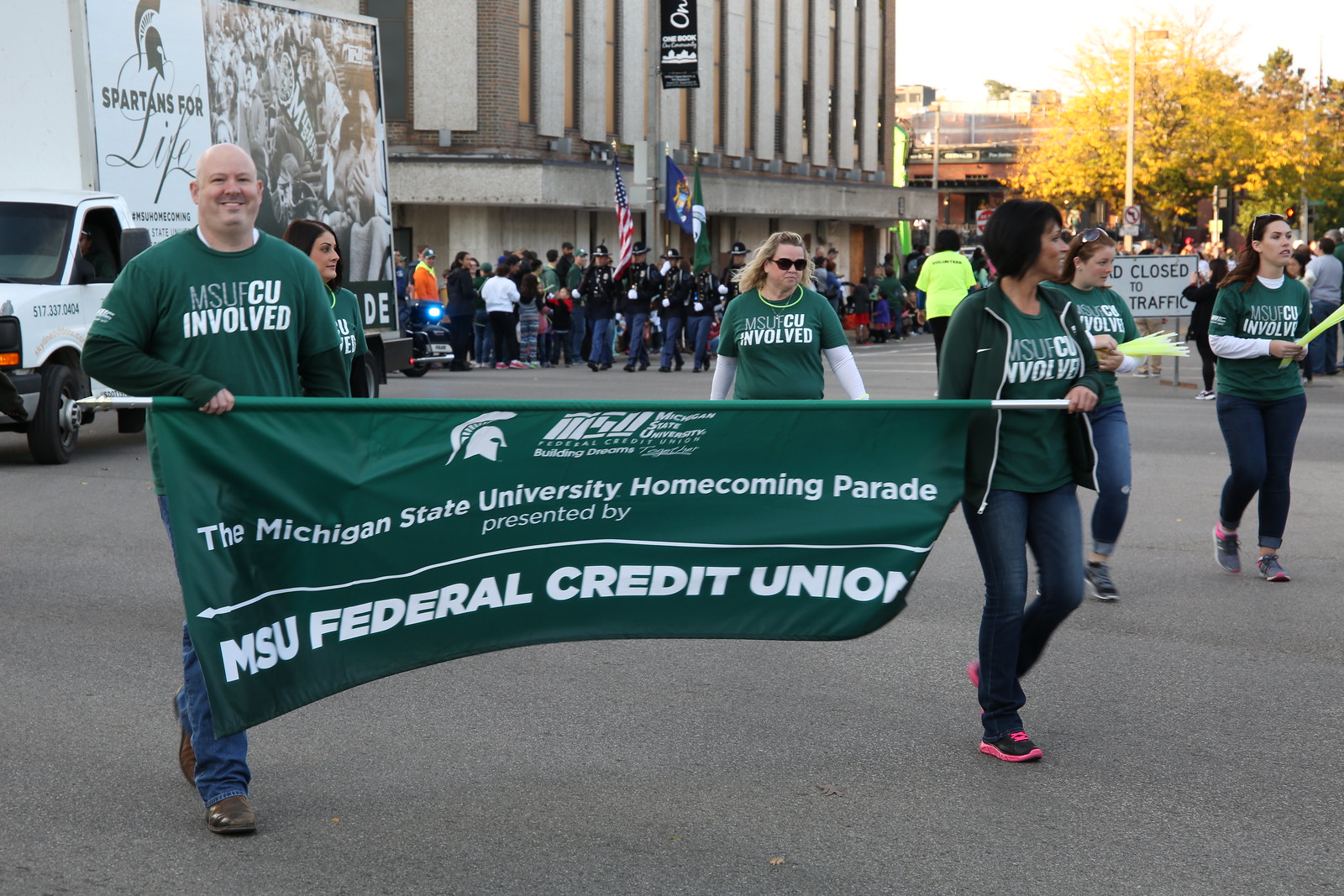In this landscape-oriented color photograph, a group of participants is marching in a parade along a blacktop city street, prominently carrying a dark green banner. The banner, held by a man on the left and a woman on the right, reads "The Michigan State University Homecoming Parade presented by MSU Federal Credit Union" in bold white text, accompanied by a Spartan helmet logo at the top. Both banner carriers are dressed in green t-shirts with the logo "MSU FCU Involved" and are wearing jeans, with layered long-sleeved shirts underneath. The man is balding, and the woman has long black hair and brown skin.

Behind them, several other individuals wearing the same green t-shirts and jeans are visible. To the left, a large white truck bearing a "Spartans for Life" banner and a photo of people is seen. The background features older multi-story brownstone buildings and a large concrete building with long rectangular windows. Behind the parade participants, there are people lined up on both sides of the street, along with police officers in uniform marching with the American and Michigan state flags. The upper right-hand corner of the image features trees and more buildings, capturing the essence of the urban setting.